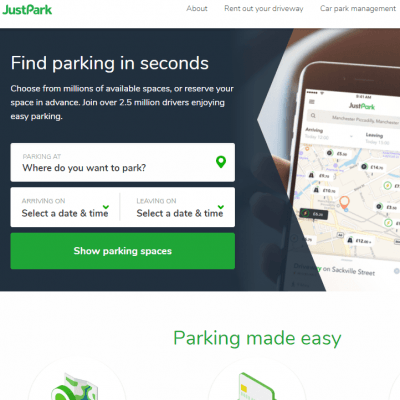The image depicts a web page for a company called JustPark, which offers convenient parking solutions. The JustPark logo is styled as a single word in green font. To the right of the logo, the navigation menu includes options for "About," "Rent Out Your Driveway," and "Car Park Management."

Central to the webpage is a prominent black box featuring white text that reads: "Find Parking in Seconds, Choose from Millions of Available Spaces, Reserve Your Space in Advance, Join Over 2.5 Million Drivers, Enjoying Easy Park." Below this box are three input fields designed for user interaction. The first field is white and prompts: "Parking At, Where Do You Want to Park?" The second white field is segmented for date and time input, labeled "Arriving On, Select a Date or Time," and "Leaving On, Select a Date and Time." The last box is green with white text stating, "Show Parking Spaces."

To the right of the input fields, there is an image of a smartphone displaying a map and navigation instructions related to JustPark. The phone is held by a hand, with three fingers visible. Below this setup, there's a green-font heading that reads "Parking Made Easy," accompanied by partially visible marketing photos that are not distinctly identifiable.